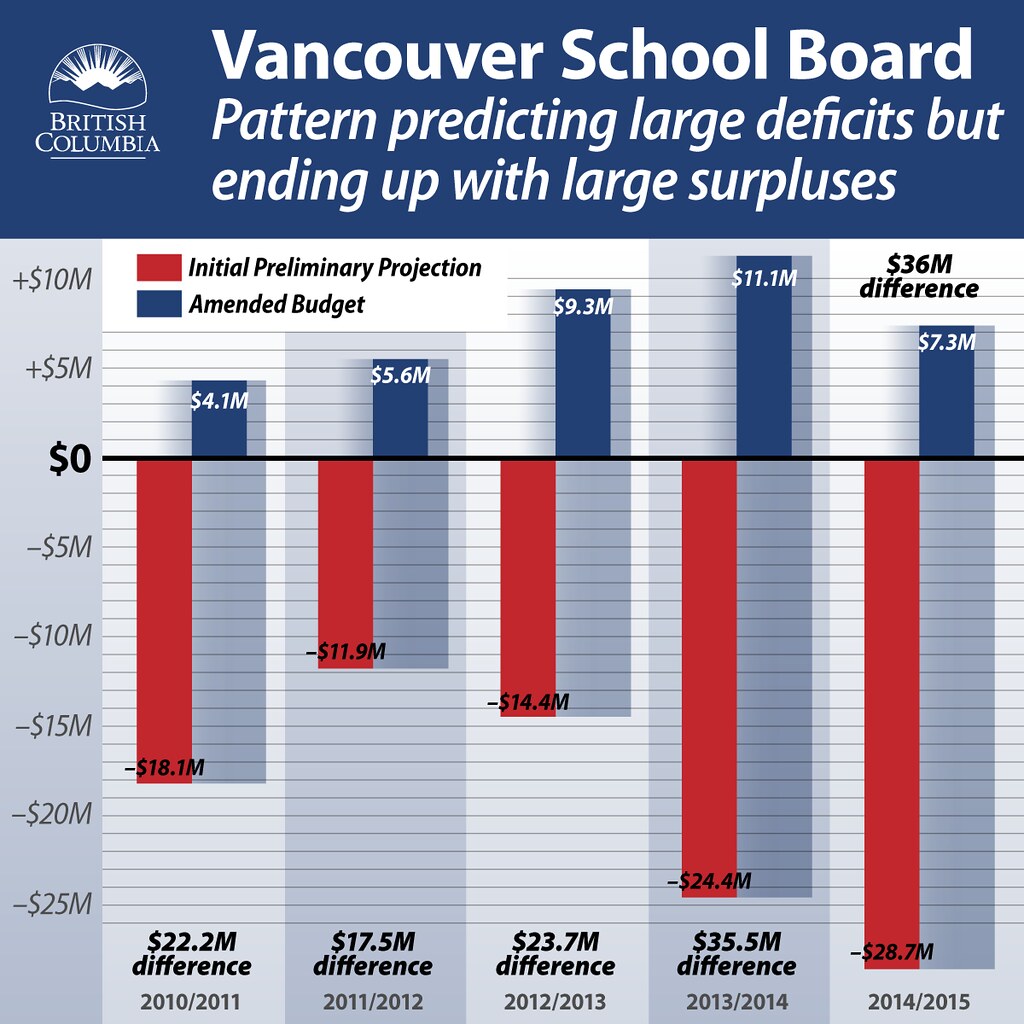This infographic presents a bar graph depicting the Vancouver School Board's financial outcomes from 2010 to 2015. At the top, a thick dark blue header features the British Columbia logo, displaying a mountain range with a sunrise. Adjacent text in white reads, "Vancouver School Board pattern predicting large deficits but ending up with large surpluses."

The graph uses red bars to represent initial preliminary projections and blue bars for amended budgets, with financial data ranging from negative $25 million to positive $10 million. Vertical labels on the left show these values in increments of 5 million, with a bold horizontal line at the zero mark.

Five bar graphs track financial differences over five fiscal years:

1. **2010-2011:** A $22.2 million difference, red in the negatives and blue in the positives.
2. **2011-2012:** A $17.5 million difference.
3. **2012-2013:** A $23.7 million difference.
4. **2013-2014:** A $35.5 million difference.
5. **2014-2015:** The largest, a $36 million difference.

Overall, the infographic conveys a consistent pattern of initial deficit projections (red) ultimately resulting in considerable surpluses (blue) for each analyzed year.